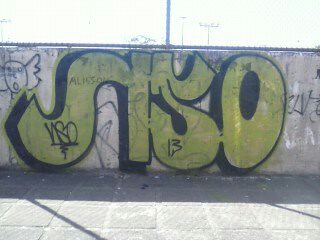The image captures a vibrant outdoor scene, centered around a stone wall adorned with various graffiti. Dominating the middle of the wall, large lime green letters spell out "S-I... something akin to an S or Y, followed by an O." The upper left-hand corner features an angel-like figure spray-painted in black. The wall is located on a paved area comprised of gray stone squares, suitable for walking. In the background, the light-colored, nearly white sky appears cloudless, and distant streetlights and power poles are faintly visible, providing an urban backdrop.